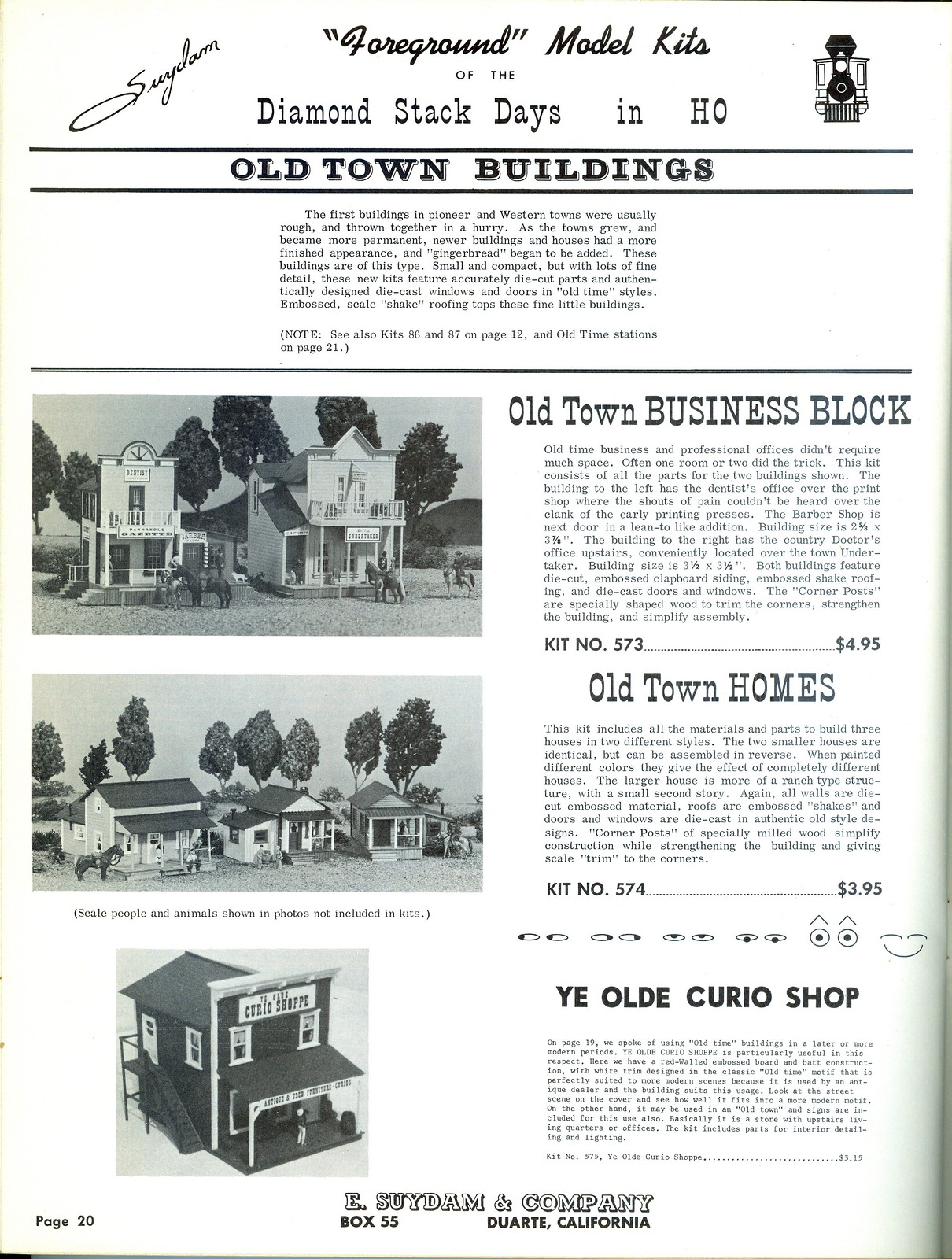The image showcases a vintage pamphlet, predominantly white with black lettering, advertising "Foreground Model Kits of the Diamondstack Days in HO." The title "Old Town Buildings" is prominently displayed, followed by a descriptive paragraph. Down the left side are three black-and-white images of various buildings, each accompanied by a detailed description on the right. 

The first image is labeled "Old Town Business Block" with accompanying explanatory text. The second is "Old Town Homes," followed by relevant details. The third image features "Ye Olde Curio Shop." The corresponding descriptions provide kit numbers and prices; for instance, "Old Town Business Block - kit number 573 for $4.95" and "Old Town Homes - kit number 574 for $3.95." 

A black locomotive emblem adorns the top right corner. At the bottom of the pamphlet, "E. Suydam & Company, Duarte, California" is clearly printed, marking the producer. Note that some text appears in cursive and parts of the pamphlet hint at late 19th-century Wild West architectural styles intended for model kits.